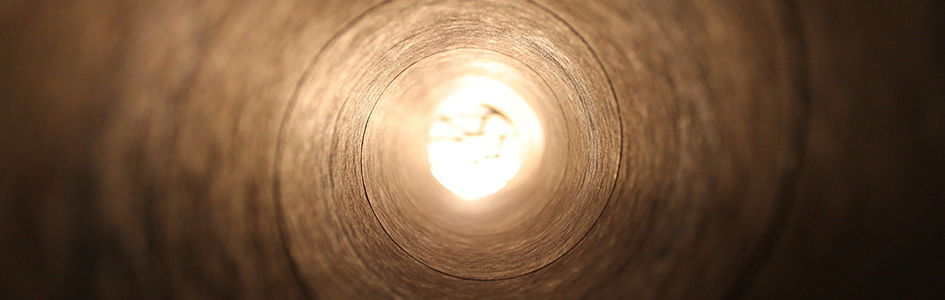The photograph captures the interior of a cylindrical tunnel with a textured, spiral-patterned wall predominantly in shades of brown, accented by lighter brown or black spiral lines. This cylindrical structure, potentially made of cardboard or concrete, extends linearly and tapers off towards a small, circular opening at the far end. Through this opening, a bright, white-yellowish light can be seen, illuminating the path within. The surface inside the tunnel is rough and unpolished, adding to the overall earthy, utilitarian aesthetic. At the mouth of this tunnel, elements resembling tree branches or roots can be faintly discerned, adding an organic touch to the otherwise stark and industrial composition. The image conveys an impression of looking through the inside of a paper towel roll, with a notable interplay between shadows and light that guides the viewer's eye towards the brightly lit exit.